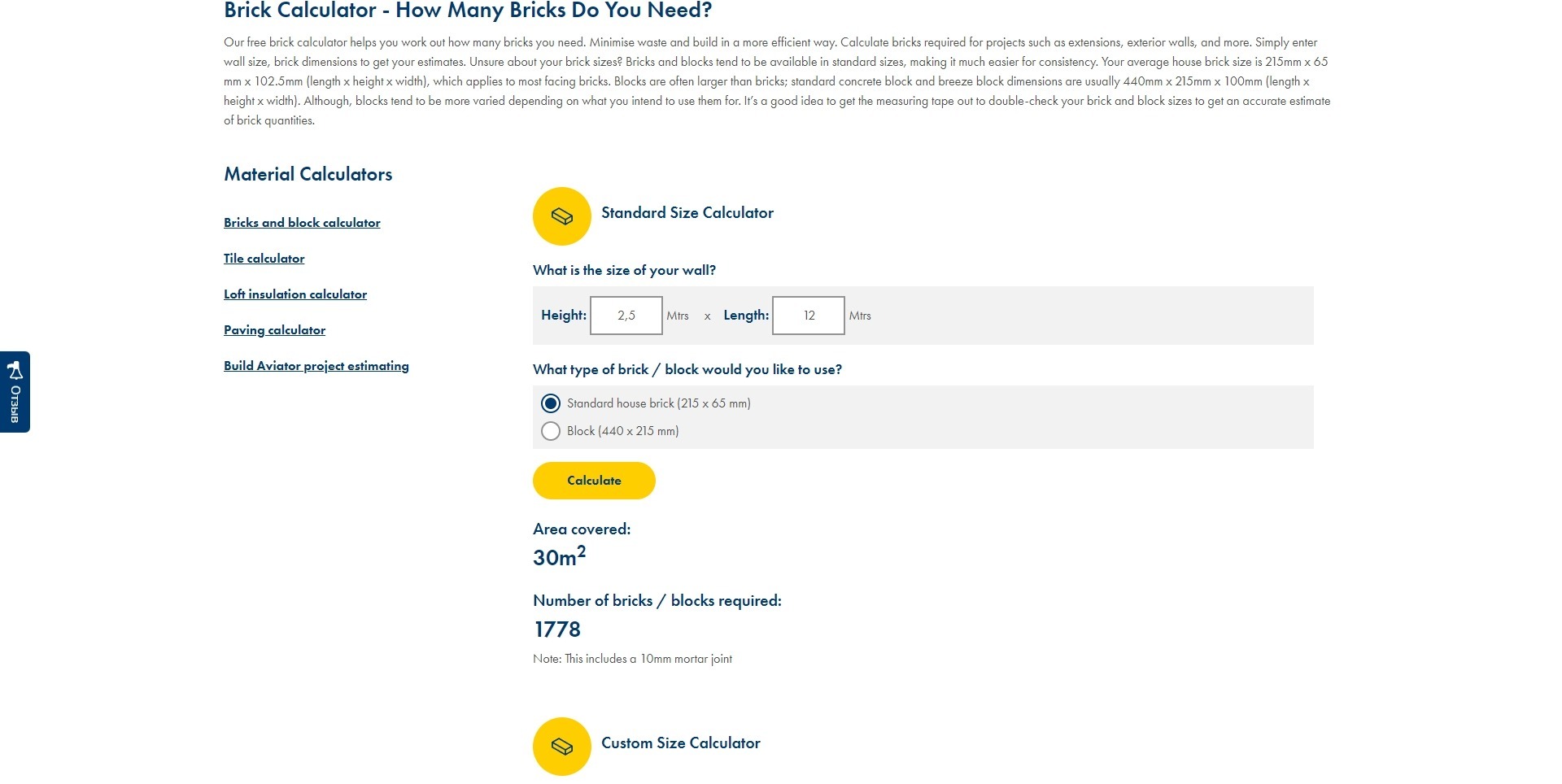"Introducing the Brick Calculator: a versatile and free tool to help you determine the exact number of bricks required for your upcoming projects. The calculator simplifies planning for exterior walls by allowing you to input specific dimensions, ensuring that you choose the correct brick sizes for uniformity and consistency. This handy tool supports standard brick and block sizes, such as the average house brick size, making your calculations straightforward.

The image also highlights other material calculators available, including a tile calculator. A prominent yellow circle features the call-to-action text: 'Calculate.' The interface prompts you to enter the dimensions of your wall, such as height and length (e.g., 2.5 meters by 12 meters), and select the type of brick or block, like a standard house brick (dimensions mentioned variably as 2.5 by 65 mm, 440 mm, etc.). Once you input these details, the calculator estimates the area covered—30 square meters—and precisely calculates the number of bricks or blocks required for the project, totaling 1,778 units."